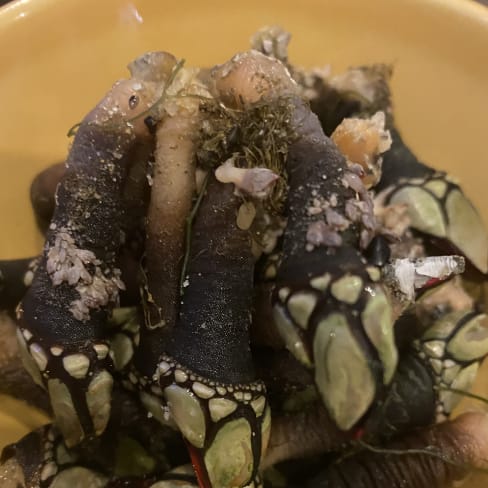The image depicts a highly detailed and complex close-up of an unidentified object or plant-like growth inside a bowl. The bowl appears to be yellow or pale orange but is mostly obscured by the contents, with only the rim faintly visible. Inside, there are numerous dark brown to almost black cylindrical structures resembling stems or roots, some of which have a light brown, hairy texture. These structures also have irregular patches of light green, grey-green, or mossy colors. The ends of these stems feature variously sized, gem-like formations in shades of yellow, green, and possibly purple, with some appearing triangular or diamond-shaped, reminiscent of animal toenails or stones. There are also hints of pink gelatinous material at the top, forming a mound shape. The overall appearance is both organic and alien, evoking a sense of curiosity and ambiguity.